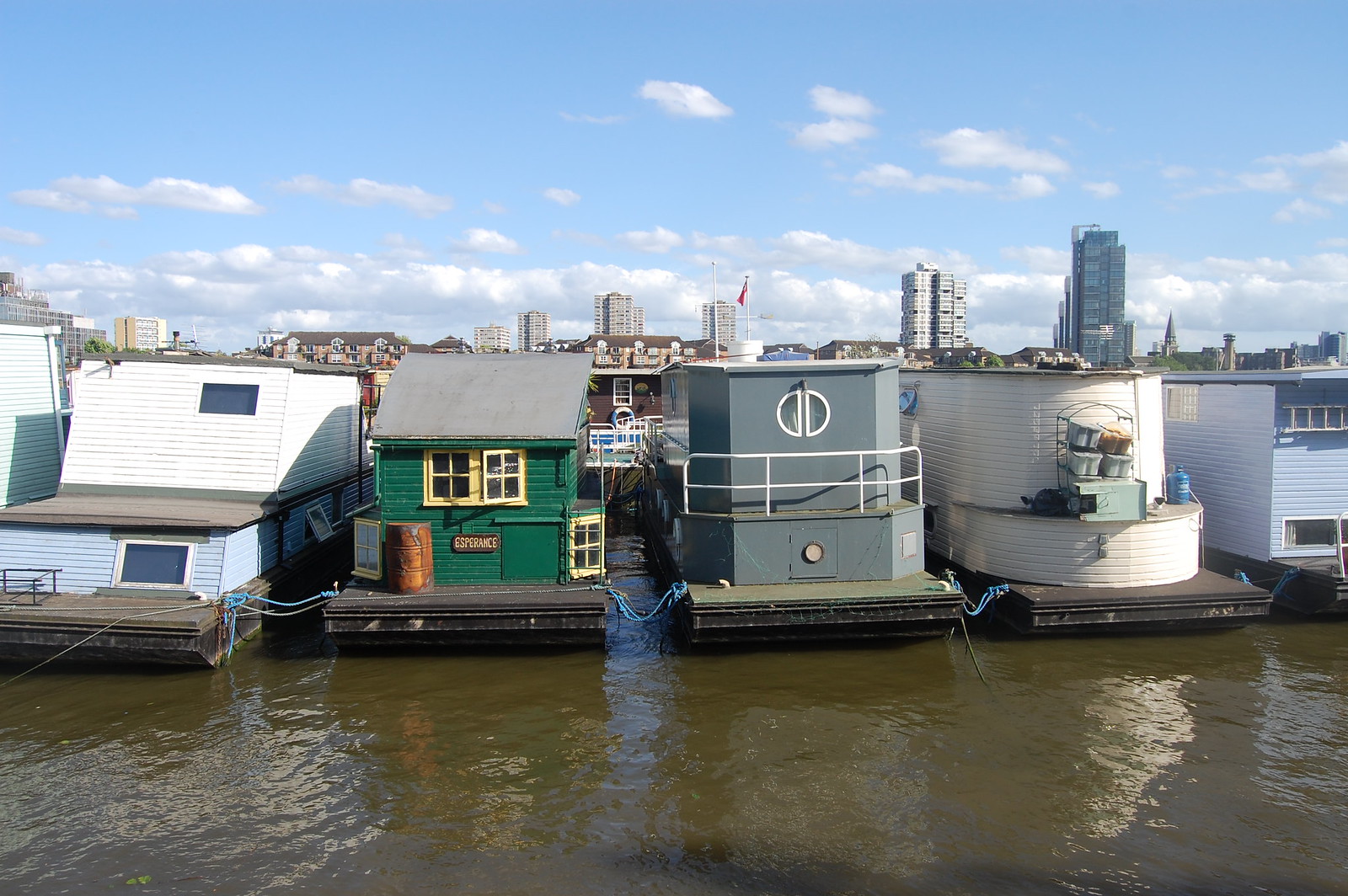This photograph, taken outdoors in a city, captures a serene waterfront scene. The image prominently features several long, narrow houseboats docked in still, chocolate-brown waters that exhibit tiny ripples. Each boat is moored with blue ropes and they stretch horizontally across the middle of the frame, spaced several feet apart from each other. The houseboats are richly detailed with multi-colored exteriors including white, gray, blue, dark green, and light blue. Specifically, one houseboat on the left displays a second story that is white with a bottom story painted blue, while another has dark green coloring with a rustic barrel and a sign that reads "Esperance."

In the backdrop, several tall city buildings rise high into the partly cloudy sky, which shows large patches of blue interspersed with puffy white and some gray clouds. A church steeple is also visible, suggesting this is a less central part of the city. The horizon is lined with these structures, hinting at the urban setting. Overall, the image juxtaposes the tranquil waterfront living with the distant urban skyline.